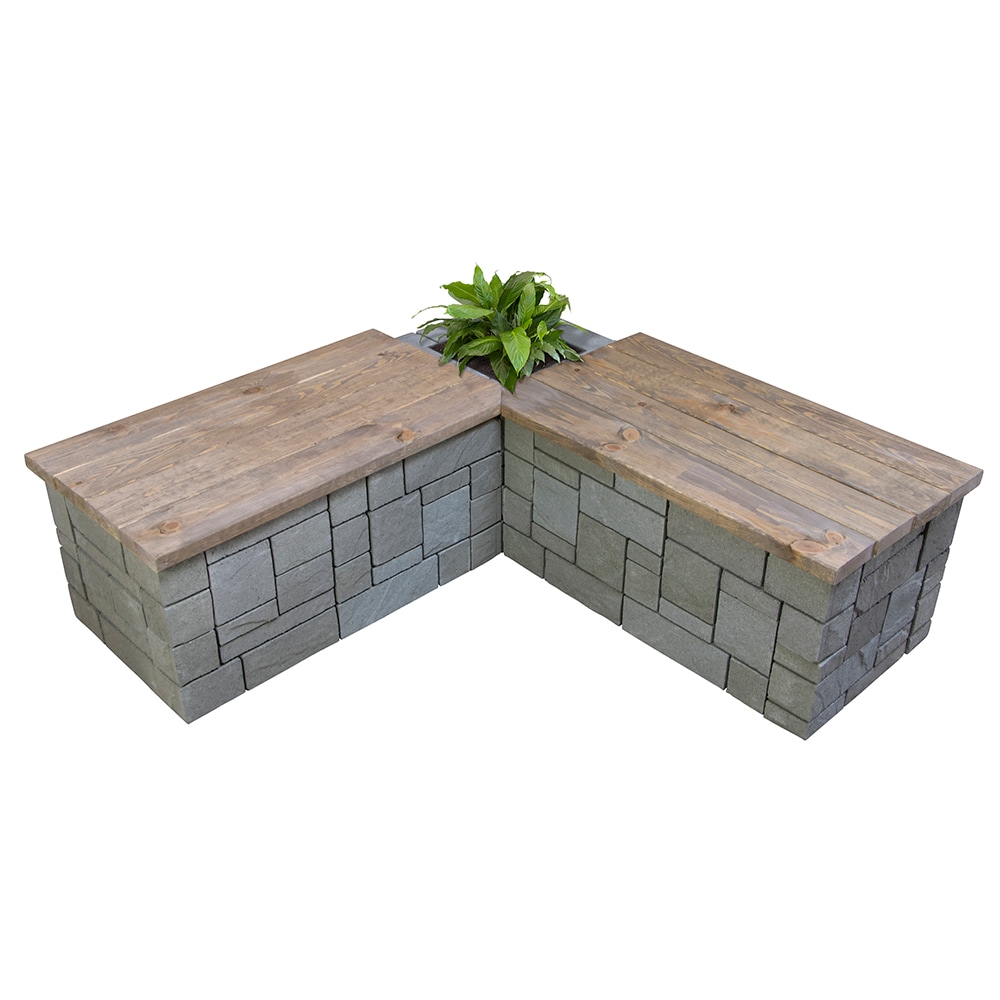The image features two identical outdoor seating benches set against an entirely white background. These benches, arranged to form an almost upside-down V shape, meet at a corner. Each bench comprises a light wood plank seating area and a base constructed from various-sized gray bricks, pieced together like a puzzle. The left bench angles upwards toward the center of the picture, with its counterpart mirroring it on the right. At the intersection where the two benches meet, there is an integrated planter containing a green leafy plant, adding a touch of nature to the L-shaped configuration of the benches.